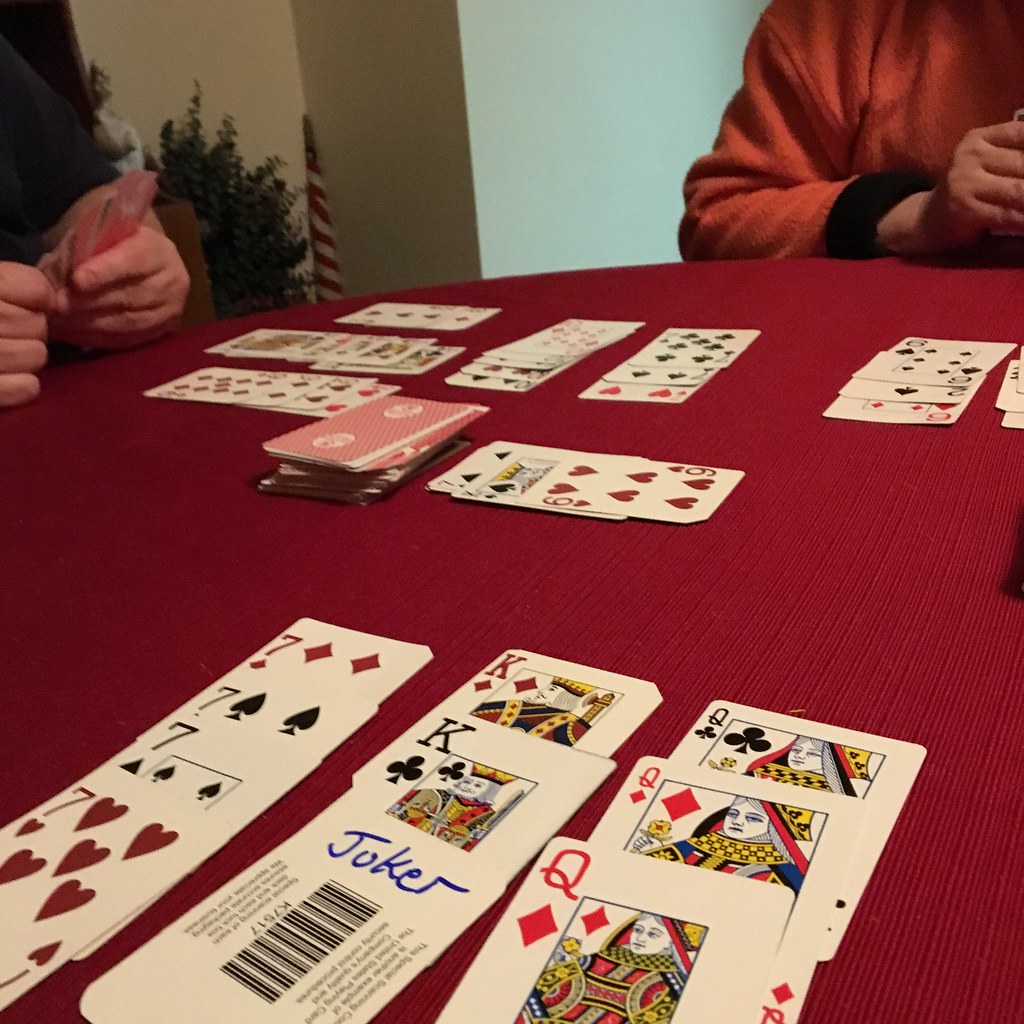In this captivating photo of a poker game, two players are engrossed in their hands. The player on the left holds a set of red playing cards, their fingers tightly gripping the deck. Diagonally across the table, another player is visible, clad in an orange sweatshirt with darker, black cuffs at the end of the sleeves. The table itself is a vibrant red, strewn with an intriguing assortment of playing cards.

In the foreground, a variety of cards are prominently displayed: sevens of diamonds and spades, additional spades, and red hearts. In the central column, the king of diamonds and the king of clubs flank a card marked as the blue joker, identifiable by its barcode. To the right, the queen of spades, queen of clubs, and another queen of diamonds are in view. Adding to the intensity of the game, a stack of cards rests conspicuously in the middle of the table, hinting at the ongoing strategies and decisions yet to unfold.